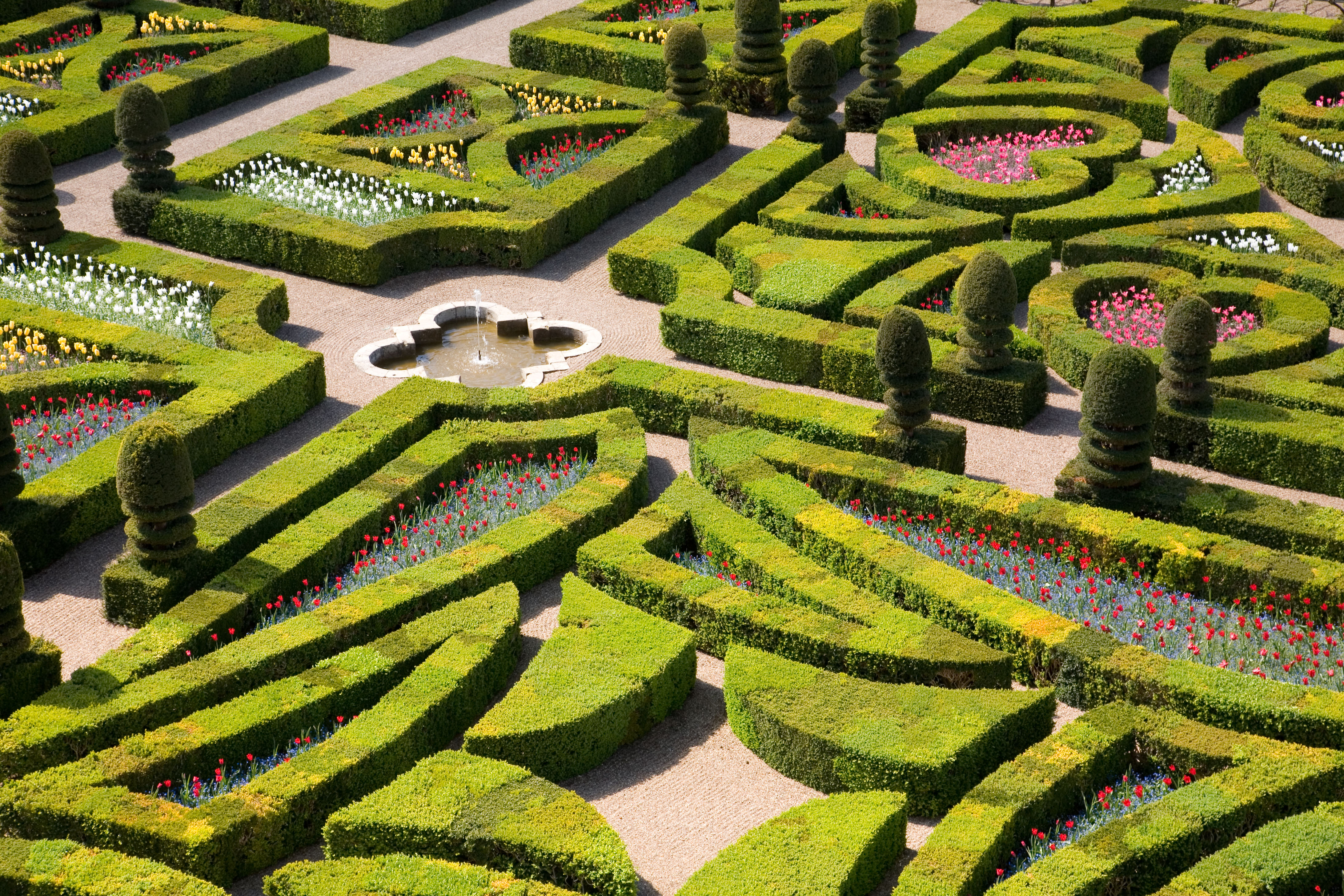This image is an overhead photograph of a meticulously manicured garden, evocative of formal and stylized old English landscapes, possibly reminiscent of Versailles. The garden is divided into several square and rectangular sections with precisely trimmed hedges in sophisticated, intricate patterns, including elongated, curved shapes resembling horns or commas, and triangular forms that appear like delicate sails. Within the hedged designs are colorful flower beds featuring red, pink, white, and yellow blooms.

At the heart of the garden lies a central fountain, adorned with decorative scrollwork, surrounded by an orderly arrangement of hedges and pathways constructed of fine pea gravel or light tan bricks. Some hedges form distinctive designs such as hearts, each harboring clusters of purple and pink flowers. Other sections include overarching, curved shapes and domed areas that extend outward, contributing to the garden's elaborate aesthetic.

Pathways meander through the garden, intersecting at various points and inviting exploration. The walkways are lined with dark green, rounded, or conical-shaped shrubs at their entrance, adding vertical interest and formal symmetry. The detailed and formalized garden presents an almost overwhelming pattern to the viewer's eye, with every element contributing to a harmonious yet complex visual feast.